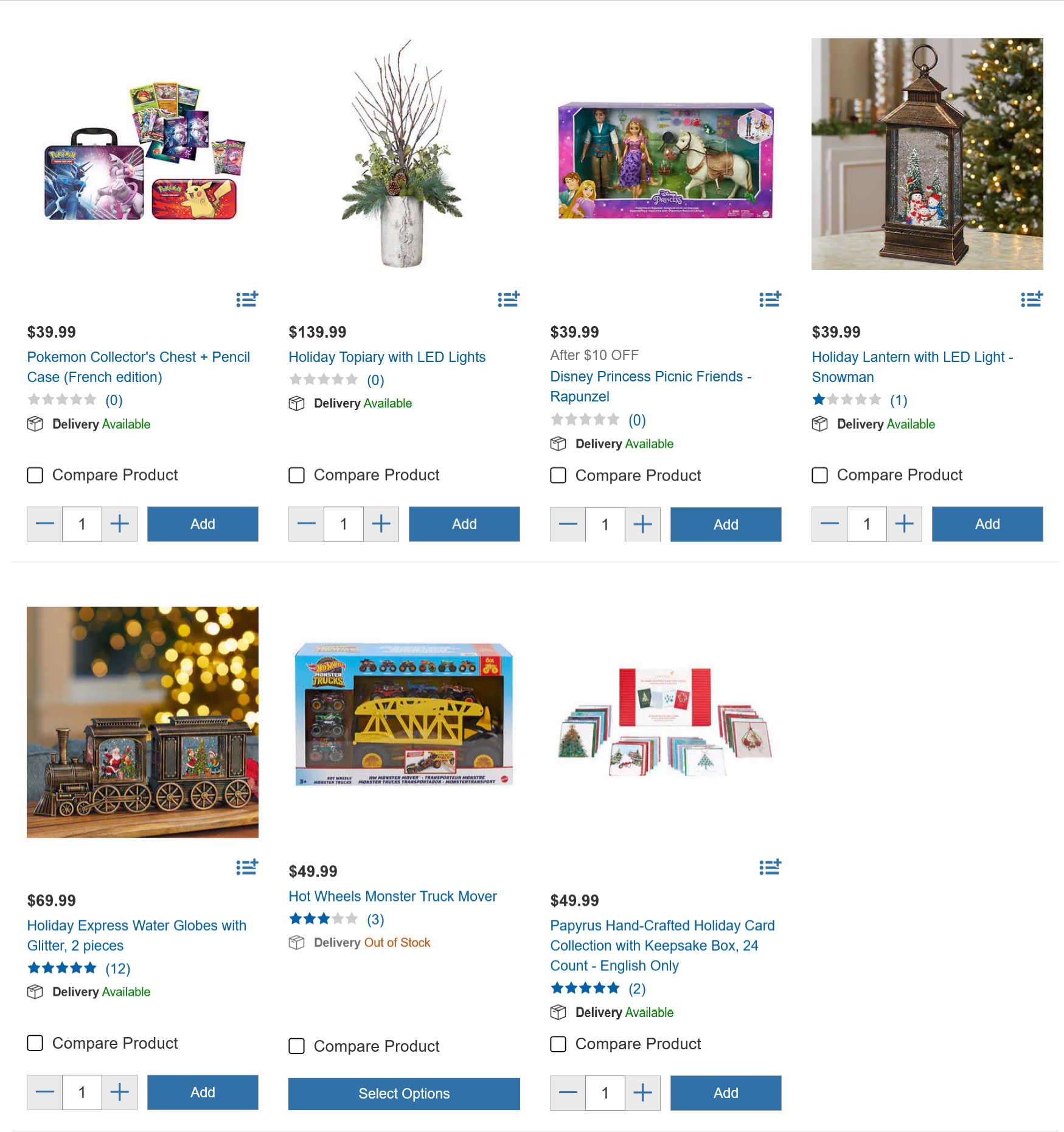This image showcases a desktop view of a holiday-themed e-commerce website, featuring an array of products geared towards Christmas presents and accessories. The layout consists of a total of seven items arranged across two rows; the top row contains four products, while the bottom row features three. Each product has options for adding or removing items, adding them to the cart, or selecting additional customization options. Here's a detailed breakdown of the items displayed:

- **Top Left ($39.99)**: A French edition Pokémon Collector's Chest and Pencil Case, with delivery available.
  
- **Second Item ($139.99)**: An LED-lit Holiday Topiary, also available for delivery.
  
- **Third Item ($39.99)**: Disney Princess Picnic Friends Rapunzel set, now at a discounted price of $39.99 after a $10 reduction. This set includes small dolls of Rapunzel and Flynn Rider from Tangled, along with Maximus the horse. Delivery is available for this item.
  
- **Fourth Item ($39.99)**: A Holiday Lantern with LED lights, designed as a snowman lantern snow globe. This item has received a single one-star review and is available for delivery.

- **Bottom Row Left ($69.99)**: Holiday Express Water Globes with Glitter, a two-piece train set featuring Santa in one globe and what appears to be elves in the second globe. This product boasts 12 five-star reviews and is available for delivery.
  
- **Second Item on Bottom Row ($49.99 - Out of Stock)**: A Hot Wheels Monster Truck Mover, resembling a large construction vehicle capable of holding various cars. This item is currently out of stock.

- **Bottom Right ($49.99)**: A Papyrus Handcrafted Holiday Card Collection with a keepsake box, containing 24 holiday cards featuring snowmen, Christmas trees, and other festive designs. This English-only collection has garnered two five-star reviews and is available for delivery.

This comprehensive webpage offers a selection of children's toys, decor, and holiday-themed items, serving as a convenient destination for Christmas shopping.